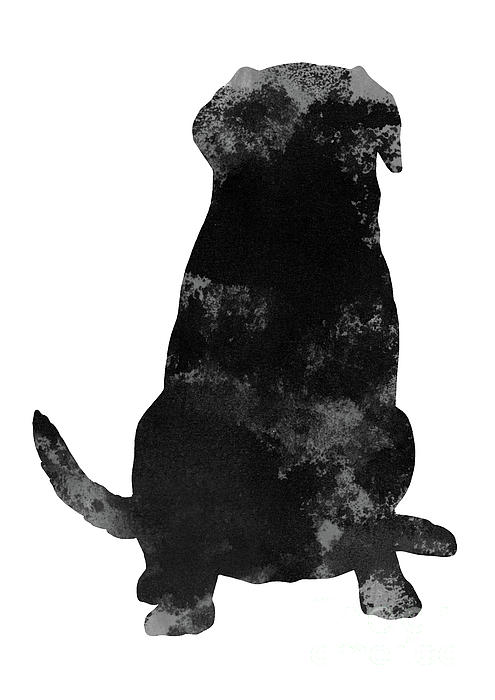The image appears to be an artistic representation of a dog, portrayed as a silhouette. The outline of the dog is clearly defined with distinguishable ears and a tail pointing to the left. The dog is depicted in a seated position, with its back legs folded underneath and front legs extending forward. The silhouette is primarily composed of black and grey splotches, resembling a sponged effect within the dog outline. The black color dominates, while lighter grey areas are more visible around the head and ear region, as well as near the tail and the feet. The background remains plain white, enhancing the contrast of the dog’s silhouette. This artistic piece evokes the appearance of a dog without detailing its facial features, focusing instead on the contour and posture of the animal.